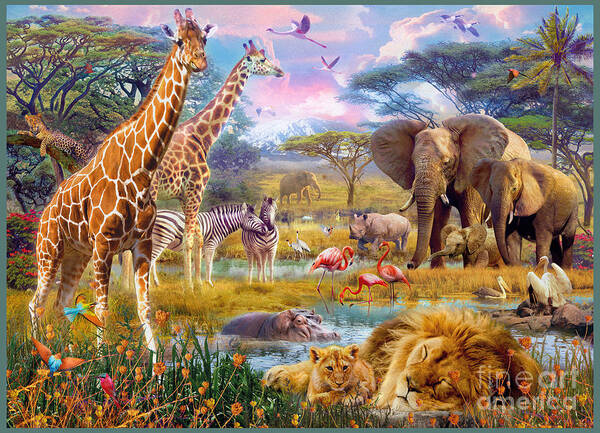This vivid painting captures a bustling scene of wildlife in a picturesque setting, featuring a blend of realistic and slightly futuristic elements. The sky is a mesmerizing gradient of pinks and blues with a few puffy clouds, adorned by flying waterfowl with long legs and big wings. In the foreground, two large giraffes stand majestically on the left, while a lion and its cub rest peacefully at the bottom right amidst a bed of blooming flowers. Scattered across the scene, there are multiple ponds; the larger one in the front hosts a hippopotamus and three pink flamingos, one of which is dipping its head into the water, while a pelican perches on a nearby rock. Two zebras nuzzle affectionately near the smaller pond in the back, beside another hippopotamus. On the far right, a pair of elephants accompany a baby elephant, and two birds rest on stones nearby. In the distance, more trees frame the scene, and a leopard lounges on a tree branch to the left. A rhinoceros and more birds add to the lively display of animals. There is even a mention of fineartamerica.com at the bottom right, hinting at the possible origin of this detailed and dynamic composition, set against a mountain backdrop that completes this stunning depiction of nature's splendor.